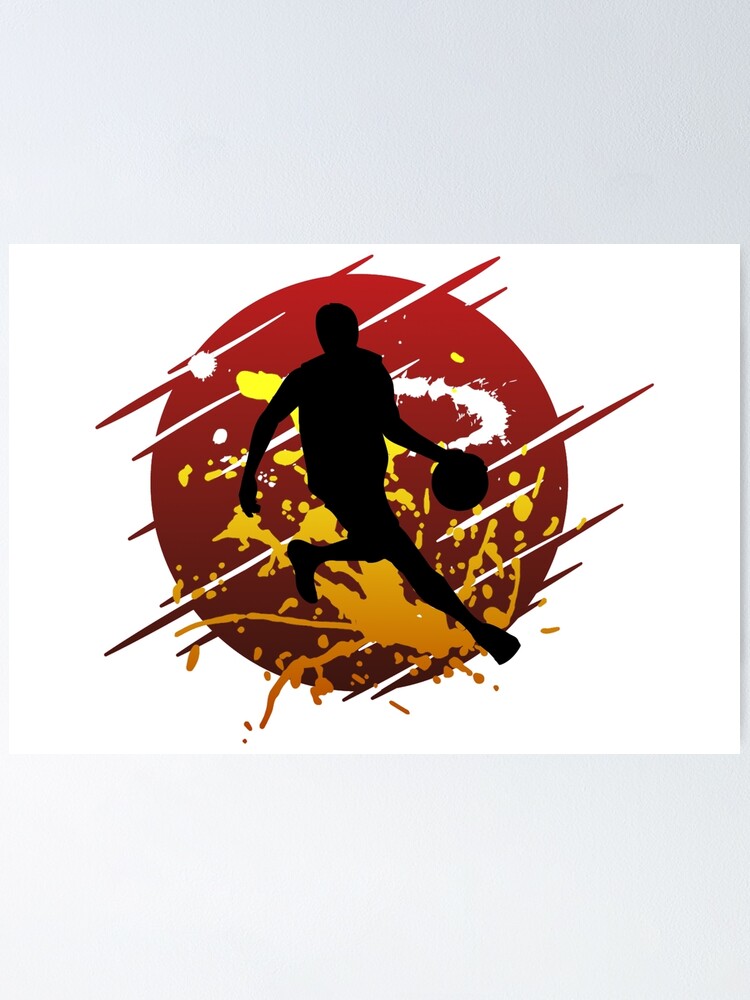The image is a digitally synthesized or hand-drawn poster in a logo-like style, set against a white background. Dominating the center is a red circle with a gradient transitioning from a lighter red at the top to a darker red at the bottom. This circle features white streaks, suggesting movement or speed. Layered over this red circle is a dynamic black silhouette of a male basketball player. The player is poised in mid-motion, with one leg extended to the right and the other leg slightly lifted toward the left side of the image. He appears to be dribbling a basketball with his right hand. Behind the silhouette, there is a vibrant graffiti-style paint splatter in shades of white, yellow, and orange, further enhancing the sense of energy and action. The player's attire is defined by the silhouette, showing him in shorts and a jersey, and the overall composition is lively and vibrant, capturing the dynamic essence of basketball.